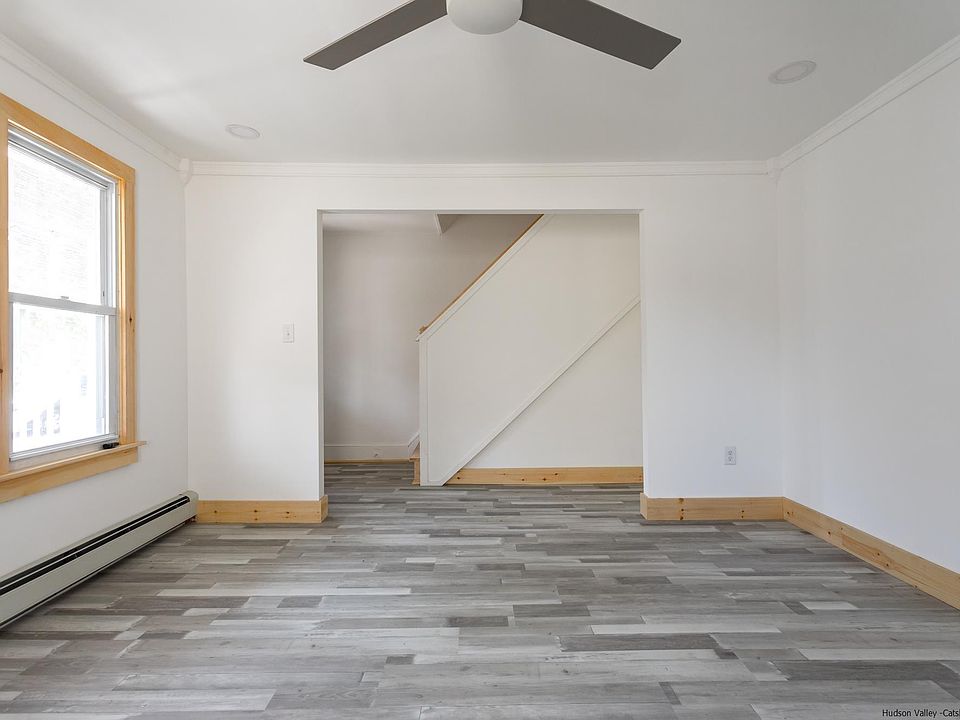The photograph depicts an empty, contemporary room with a clean, modern aesthetic. All walls and the ceiling are pristine white, creating a bright and airy atmosphere. The floor features a medium-gray, wood-patterned finish, enhancing the room's modern look. Baseboards and window frames are made from light, unstained wood, giving a subtle yellow hue that contrasts gently with the white walls. A baseboard heater is positioned beneath a window on the left side, which is illuminated by abundant daylight from outside.

A stylish ceiling fan with two large, gray blades and a central white light fixture is mounted on the ceiling, accompanied by two recessed lights that provide additional illumination. The room extends into a hall and a staircase area, visible through a large cutout on one end of the room. Though the stairs themselves are not visible, the upward ascent of the staircase is indicated by a steeply angled banister. This open, inviting space, devoid of furniture, appears to be staged for a real estate or rental listing.